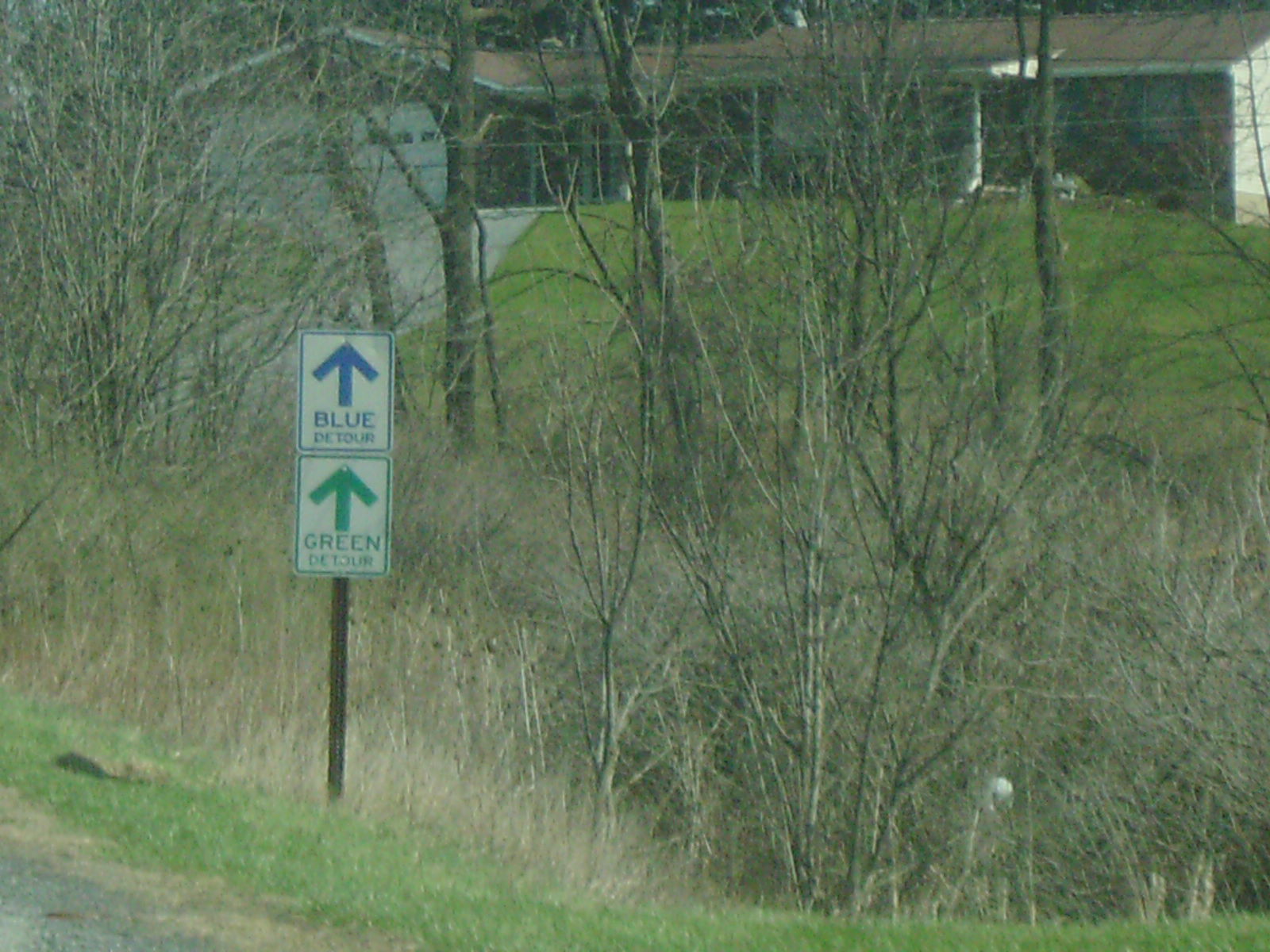A photograph taken from a road captures a small signpost positioned near the bottom left corner, suggesting the picture was taken either by a pedestrian or from a vehicle. The signpost, mounted on a wooden pole, features two directional signs. The upper sign, bordered and lettered in blue, reads "Blue Detour" with an arrow pointing upward. Below it, another sign in a green theme has a similar upward-pointing arrow and reads "Green Detour." Surrounding the signpost, the landscape is filled with barren trees devoid of leaves and a mix of overgrown grass and weeds, conveying a desolate and possibly autumnal or winter scene.